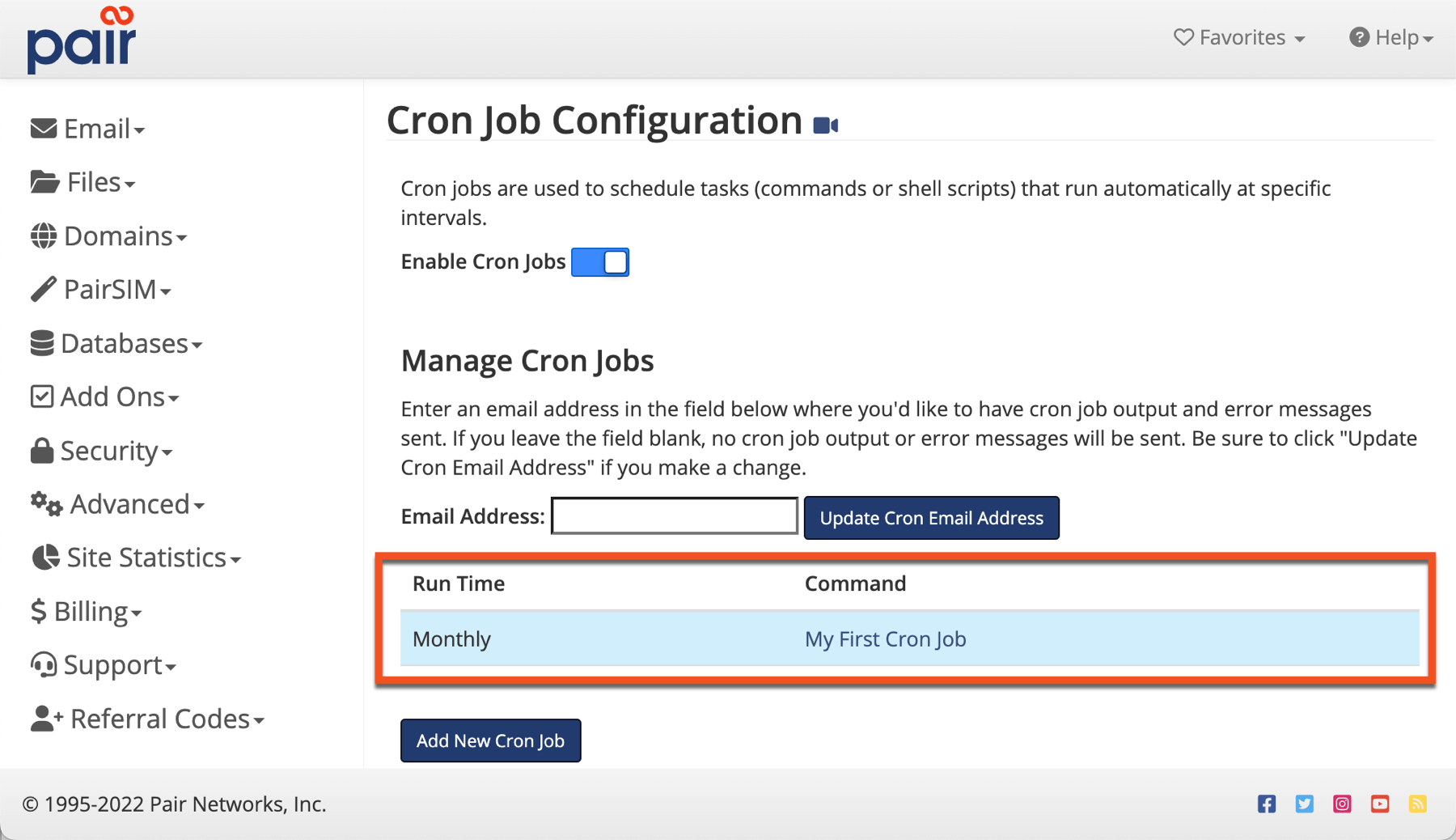This image, sourced from the PAIR website, illustrates the layout of the site's interface. At the top of the page, a gray navigation bar spans across the screen. Positioned under or within this gray bar, the upper left corner features the word "PAIR" in blue, with an infinity symbol cleverly integrated over the "A," "I," and "R" of the word.

Moving rightward along the gray bar, there are two tabs: "Favorites" and "Help." Below this navigation bar, the page transitions to a white background, which embodies the main content area.

On the left side, a vertical sidebar lists several tabs, titled: `Email`, `Files`, `Domains`, `PAIR SIM`, `Databases`, `Add-ons`, `Security`, `Advanced`, `Site Statistics`, `Billing`, `Support`, and `Referral Codes`.

Dominating the central section of the page is the header "Cron Job Configuration," which serves as the focal point of this segment. Below this header, there is a descriptive text: "Cron jobs are used to schedule tasks, commands, or shell scripts that run automatically at specific intervals." Further down, there is an "Enable" option, followed by another section labeled "Manage Cron Jobs," where details like runtime and command are displayed. This specific part of the section is distinctly highlighted with a red box, drawing attention to its importance.